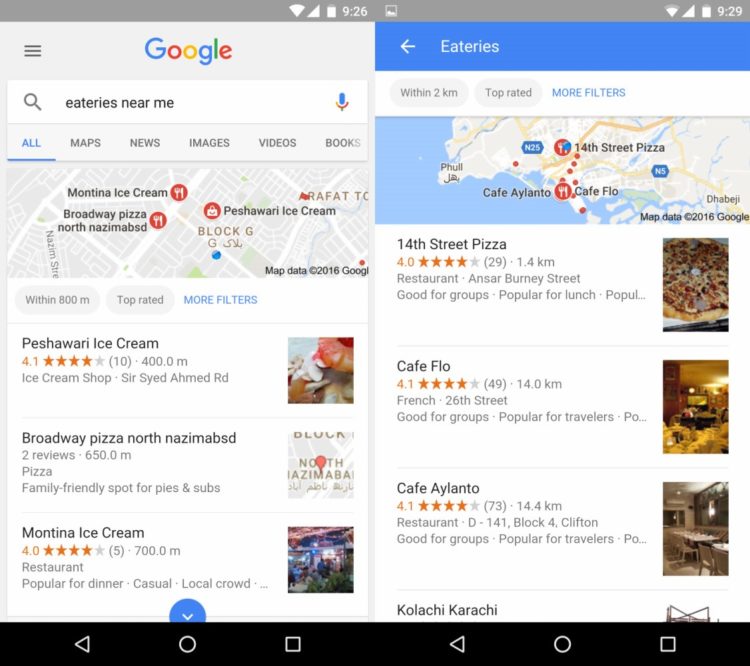The image showcases screenshots from a mobile device, likely a phone or a tablet, as indicated by the Wi-Fi notification, time, and battery symbols visible at the top of each screenshot. 

The left screenshot displays a Google search results page with the query "eateries near me" entered in the search box. Below the search box, several eateries are listed alongside a small map. The eateries visible include:
- Montina Ice Cream, which has a rating of 4 stars from 5 reviews.
- Peshari Ice Cream, rated at 4.1 stars from 10 reviews.
- Broadway Pizza in North Nazimabad, listed with 2 reviews but no star rating shown.

The right screenshot presents another Google search results page, filtered to show eateries within a 2 km radius that are top-rated. The entries include:
- 14th Street Pizza, with a rating of 4 stars from 29 reviews.
- Cafe Flow, rated at 4.1 stars from 49 reviews.
- Cafe Elanto, also rated at 4.1 stars from 73 reviews.

Both screenshots illustrate the process of using Google search to find local eateries, providing a typical view of search results including ratings and reviews for various dining options.